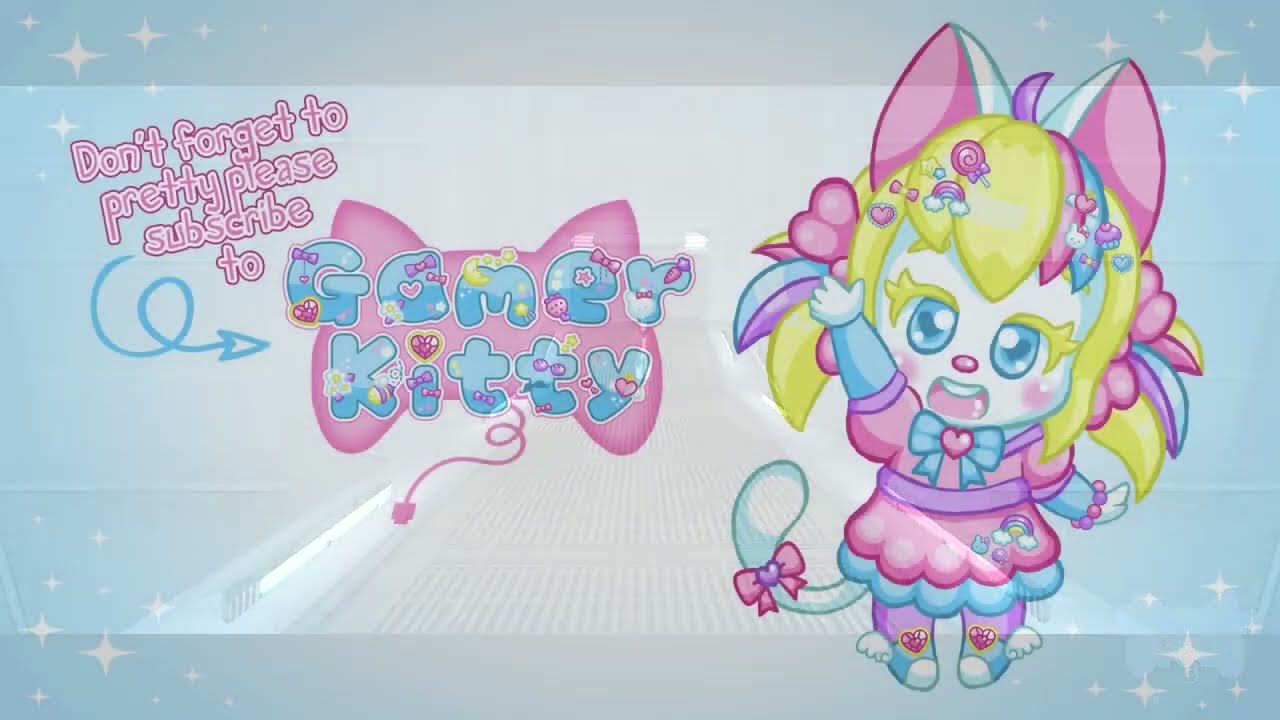The image is a pastel-colored cartoon or comic illustration featuring a composite cat-like little girl on the right side. This "Gamer Kitty" character has yellowish hair, pink cat ears, and a tail with a blue bow tied around it. She is dressed in a pink underdress with a purple and blue skirt, and a blue bow with a heart tied around her neck. Her left hand is raised as if she is waving, and her mouth is open. Gamer Kitty has blue eyes, blonde eyebrows, and is wearing winged white and blue shoes with heart accents. To the left of Gamer Kitty, there's text that reads, "Don't forget to pretty please subscribe to" with an arrow pointing to the right. The text "Gamer Kitty" is styled in a bubbly, playful font adorned with cute hearts, purple bows, and other accents, situated over a pink, game controller-shaped design. The background of the image is a light blue pastel with white stars in each corner. There's also a purple butterfly near the text. The overall scene is whimsical and inviting, with a heavy emphasis on the cute and playful elements surrounding the Gamer Kitty character.